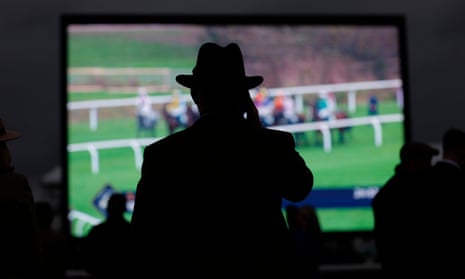In a dimly lit sports bar, a man in a suit and hat stands at the forefront, his right hand held to his ear as if talking on the phone. He gazes intently at a large screen displaying a horse race, where a cluster of horses with jockeys ride closely together on a vibrant green track flanked by white guideposts. The background reveals multiple screens, adding to the bar's ambiance, with faint silhouettes of other patrons scattered around. Notably, there's a person on the left and a couple on the right, all equally engrossed in the race. The image captures a mix of colors including greens, blues, oranges, teals, whites, and blacks, creating a vivid and bustling yet shadowy environment typical of a sports bar.